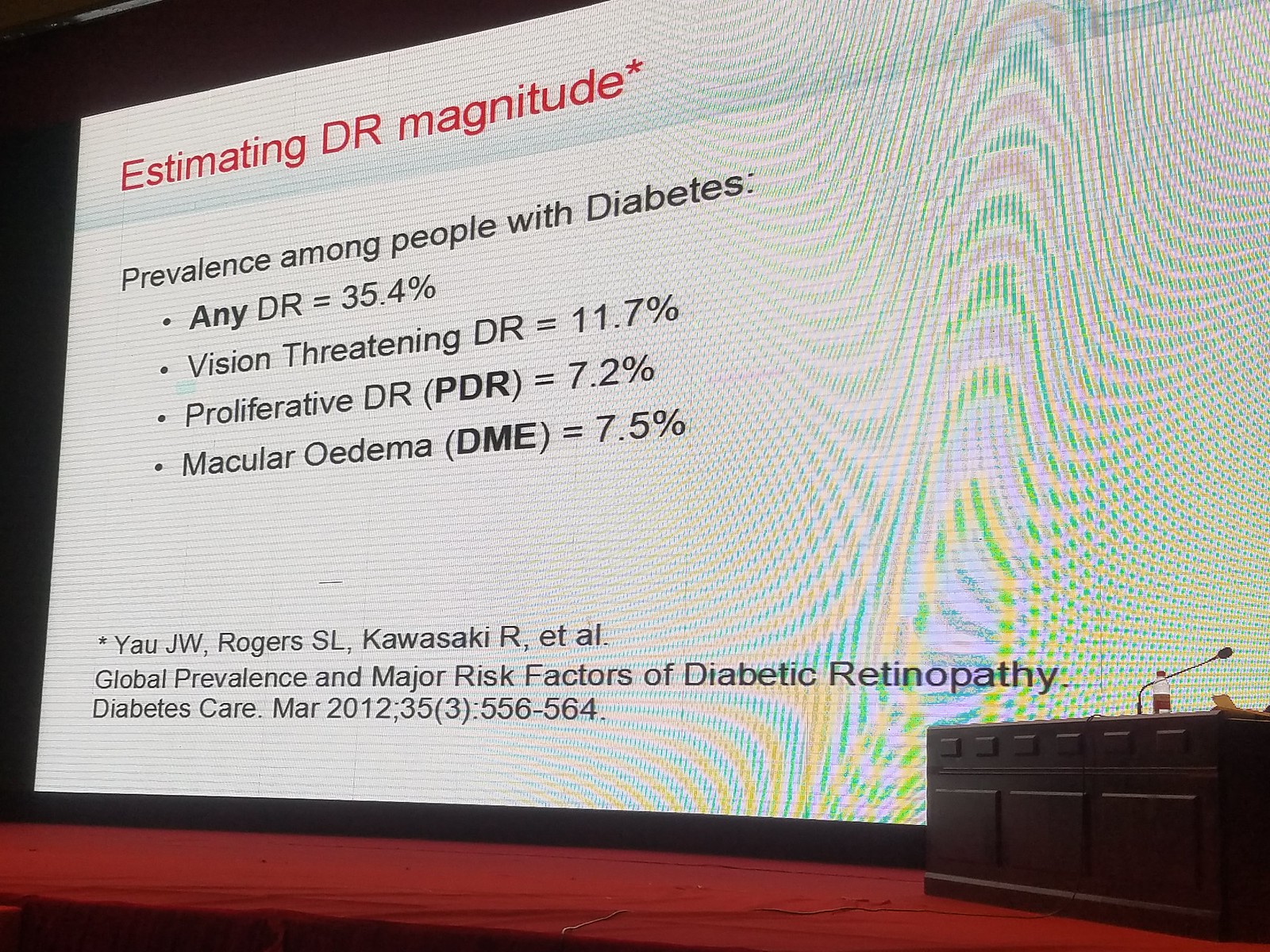The image captures a large presentation on a stage covered with a red carpet-like material, which has a slight frill along the edge. To the right, there is a brown podium with three large and six smaller panels, featuring a bent microphone pointing off-screen and a water bottle with a red cap and label. Dominating the scene is a massive projection screen displaying detailed medical information about diabetic retinopathy. The screen's title, "Estimating DR Magnitude," is in red font, followed by the subtitle, "Prevalence Among People With Diabetes" in black. Key statistics are listed: Any DR at 35.4%, Vision-threatening DR at 11.7%, Proliferative DR (PDR) at 7.2%, and Macular Edema (DME) at 7.5%. An attribution at the bottom credits Yao JW, Rogers SL, Kawasaki R, et al., with a reference to their March 2012 study in "Diabetes Care," volume 35, pages 556-564. The screen shows a pixelated rainbow pattern of blue, yellow, purple, and white hues. This presentation is evidently part of a medical conference, given its content and the sophisticated setup.